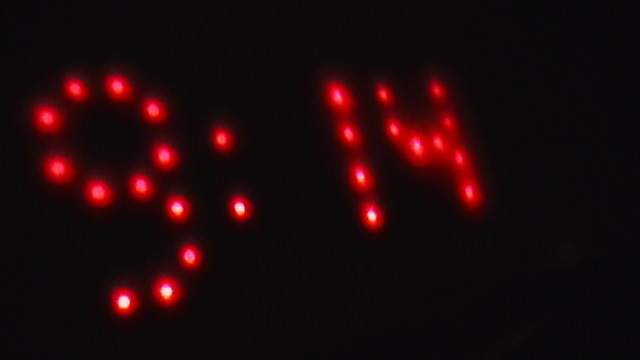The image depicts a digital clock display against a completely black background, taken in landscape mode at nighttime. The clock shows the time "9:14" with each digit formed by a series of uniformly glowing red dots. The 9 appears slightly closer and larger compared to the other numbers, while the 1 and 4 seem further away, creating a perspective effect. The dots that make up the numbers are uniformly sized, with the 1 consisting of 4 dots and the colon between the 9 and 14 made up of 2 dots. The red dots glow with a light pink hue at their center, gradually becoming darker pink and red towards the edges. The image is clear enough to read the time easily, despite not being of very high resolution. The black background is uniformly dark without any distinguishing marks, ensuring that the focus remains solely on the glowing digital time display.